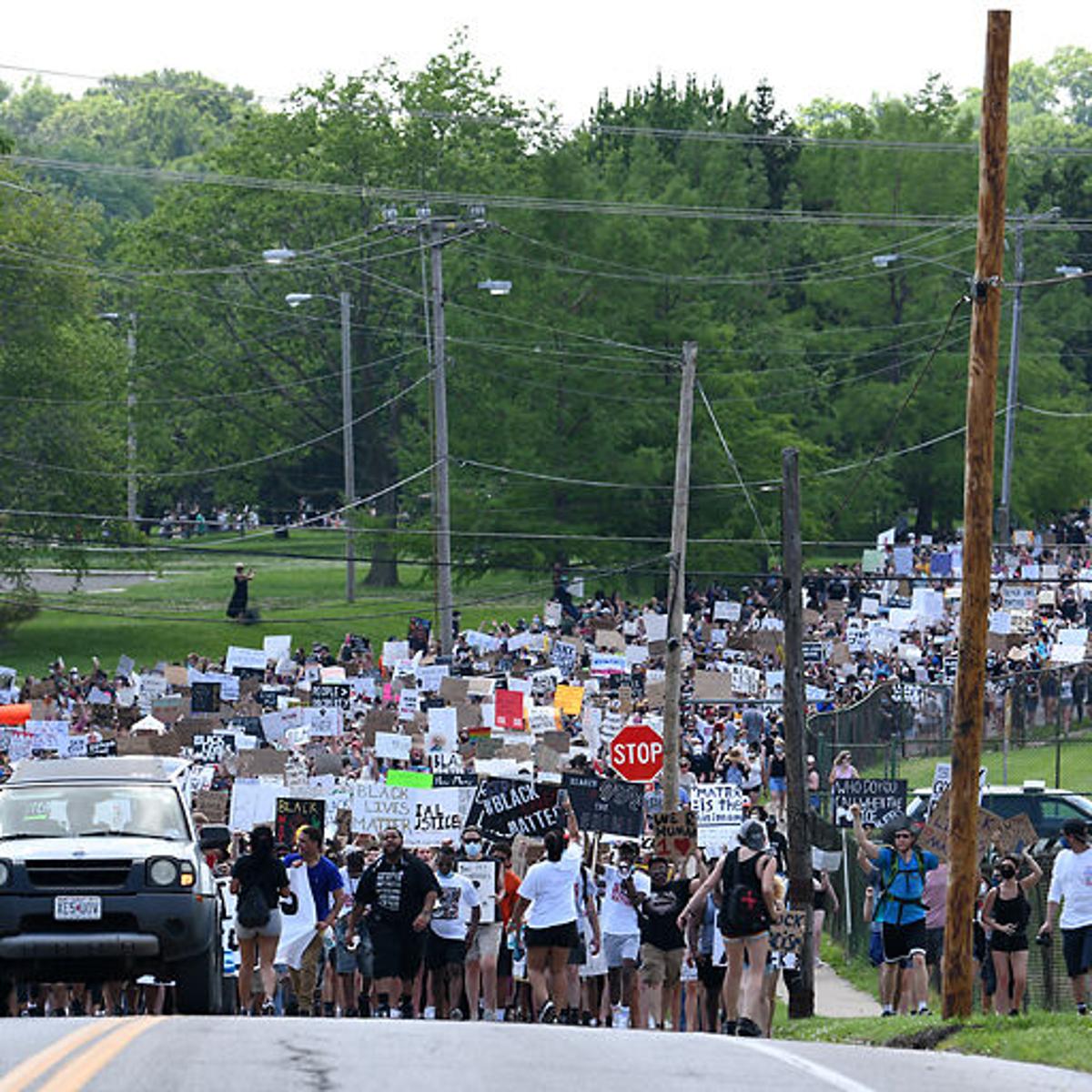The image captures a massive Black Lives Matter protest from the 2020s, set against a rural backdrop. The scene unfolds on a two-lane road densely packed with protesters extending far into the distance. In the foreground, a single white truck with a black bumper leads the march, followed by a sea of diverse participants. The crowd is a tapestry of different races and ethnicities, with many protesters holding up various signs. Prominent signs read "Black Lives Matter," "Justice," and empowerment symbols, but as the crowd stretches further back, the text on the signs becomes difficult to discern.

Above the mass of people, numerous telephone poles and power lines crisscross the sky, adding to the intricate details of the setting. The background reveals clusters of green trees surrounding the march and patches of green grass that might indicate more protesters snaking around unseen paths. People towards the front of the image are actively engaged, with some raising their arms in solidarity. The scene is set under a hazy sky, enhancing the dramatic and poignant atmosphere of this large-scale demonstration for racial justice.